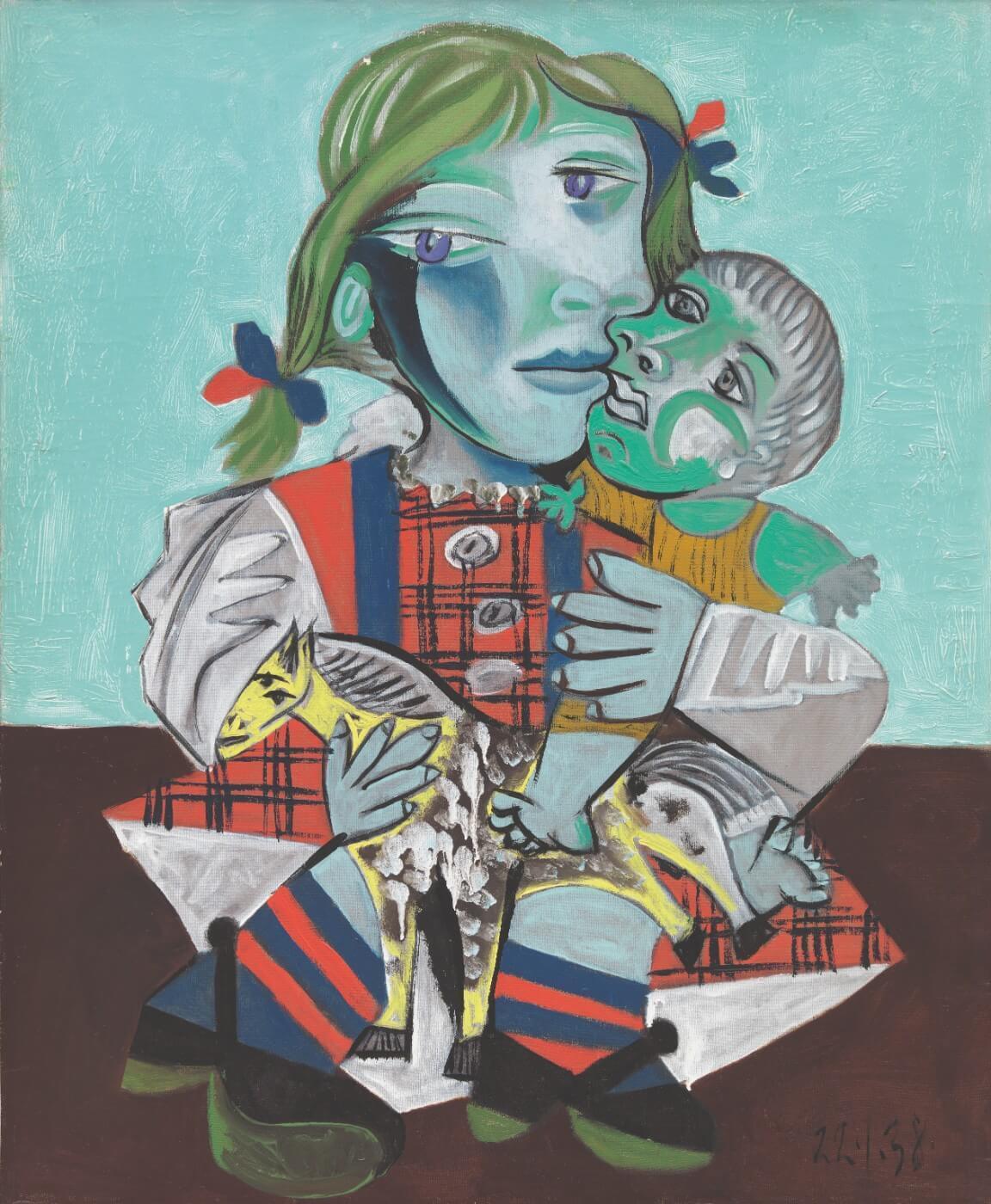This photograph captures "Pablo Picasso's 'Maya with Doll', 1938," an engaging and intricate artwork showcasing the artist's daughter, Maya, in a surreal and fragmented form. The central theme illustrates the intimate father-daughter relationship, depicting Maya holding a doll. The younger figure, Maya, is portrayed with a tank top, an unusual choice that adds to the surrealist tone of Picasso's style. Her facial features — the eyes, mouth, and nose — are distinctly Picasso, exuding an abstract and profound expression. Maya’s feet are angled in various directions, while interspersed limbs and a toy horse cross her lap, creating a dynamic and chaotic composition. Her hair is parted with shades of purple underneath, contributing to the painting’s uniqueness and distorted reality. The background is a light gray, seamlessly transitioning into a purplish-red, almost beet-colored base, enhancing the depth and emotion of the piece. This artwork is a testament to Picasso’s unique style and his deep connection with his daughter, Maya.